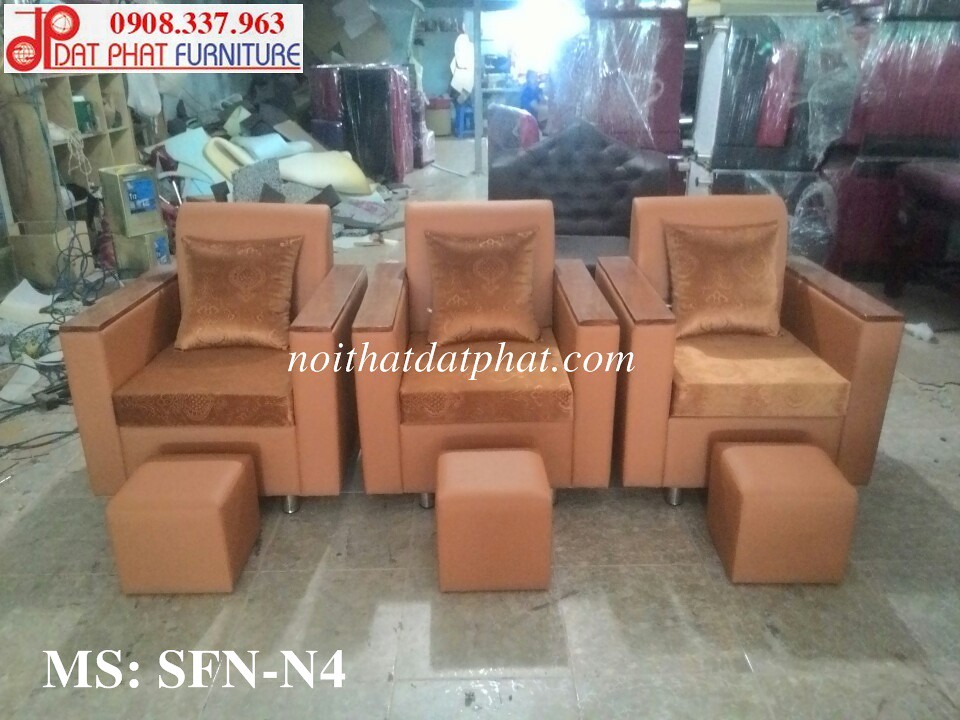This advertisement features an image of the back room of Dat Phat Furniture, possibly a handmade furniture factory, set in a large, somewhat chaotic warehouse with scattered materials such as blankets, foam, wiring, and boxes. Dominating the center of the photo, there are three finely crafted Indian-style recliners, each paired with a matching footstool. These luxurious chairs, upholstered in a light peach or bronze-orange colored fabric with a satiny, patterned texture, exemplify plush comfort with their high, flat armrests and coordinating throw pillows. The surroundings suggest this area might be where furniture is received or assembled before being displayed. Additional items in the background include cabinets, display cases, and bed headboards, some covered in plastic, all hinting at the chaotic yet productive environment. The logo "D.P." for Dat Phat Furniture, along with the website "noithatdatphat.com" and a phone number "0908 337 963," is displayed at the top-left corner, emphasizing the store's branding amidst the bustling scene.